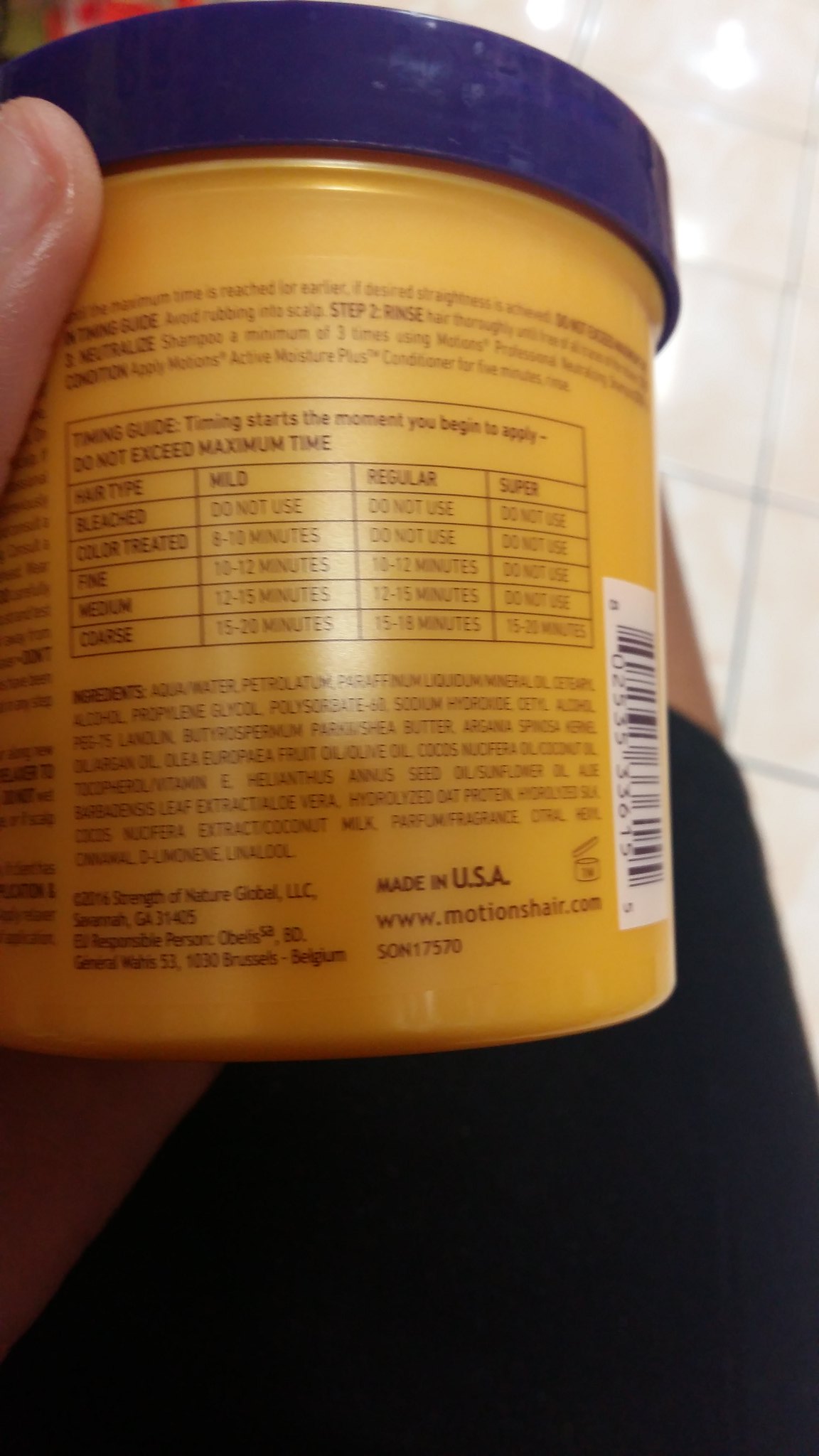In this image, a person is holding an orange plastic jar of hair straightener in front of the camera. The jar features a contrasting blue screw-on lid. The individual's thumb is visible in the top left corner of the photo, while the lower part of the frame includes a glimpse of their leg and a corner of the floor. The orange label on the jar provides detailed instructions on how to use the hair straightener, complete with a timing guide. The brand is Motion Hair, and the product is manufactured by Strength of Hair Global LLC, as indicated on the label. Additionally, the label lists ingredients, instructions for use, and a UPC code for scanning. The website motionshair.com is also printed on the label for further information.